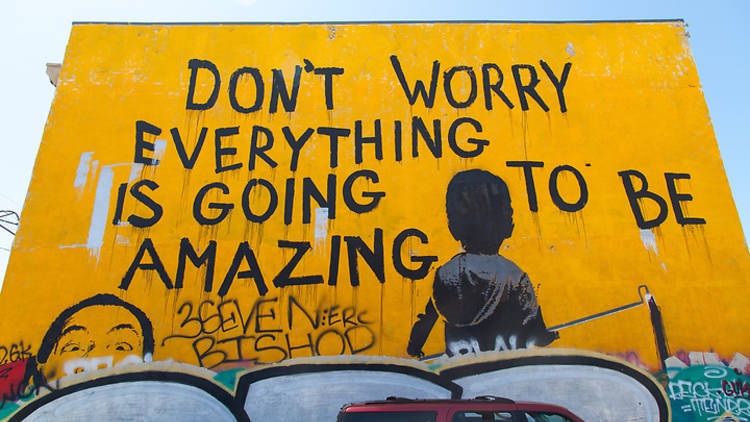The rectangular image features a tall, windowless building with a striking graffiti mural dominating its facade. The sky at the edges of the image is blue, darker on the right side than the left. The backdrop of the mural is primarily a taxi-yellow or orangish hue, and the focal point is a large, bold, black capitalized text that reads, "Don't worry, everything is going to be amazing" in four lines. Below this optimistic message, in what appears to be personal handwriting, are the characters "37ERC Bishop."

A significant element of the graffiti is the silhouette of a boy viewed from the back, dressed in a black hooded jacket, holding an extended paint roller that seems to be in the process of painting black strokes on the wall. The paint roller and boy appear as part of the artwork. To the bottom left, there is a partial, black-and-white painted illustration of the top of a man's head with dark hair, raised eyebrows, and widened eyes, stopping just above his lips. Scattered throughout the mural are some white letters and graffiti that are difficult to decipher, along with areas containing gray lines, red marks, and a small green patch with accompanying white graffiti. Additionally, the roof of a red van is visible at the bottom of the image.